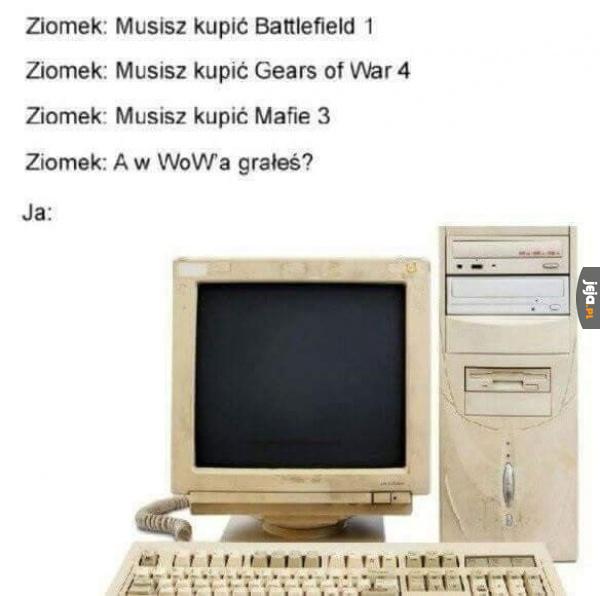The image is a meme featuring a very old, outdated computer setup against a white background. The computer appears to be from the late 80s or early 90s, characterized by its dirty, yellowing components, which were originally white. The setup includes a bulky CRT monitor, an ancient tower with a CD-ROM or possibly DVD-ROM drive, and a floppy disk drive. The keyboard is connected via an old, spiraled phone cord, further emphasizing the antiquated technology. On top of the tower, there's some text in a foreign language, which could be Russian or Czechoslovakian, listing modern video games such as Battlefield 1, Gears of War 4, Mafia 3, and World of Warcraft followed by "Gratis ja". The likely joke is that this outdated computer is hilariously inadequate for running these contemporary games.